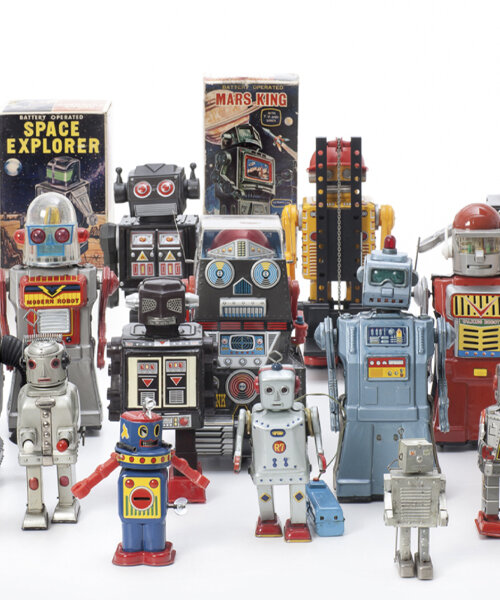The image displays a collection of vintage toy robots, likely from the 1980s or 1990s. There are around a dozen robots, with several more partially cut off on the edges of the image. The robots vary in height, seemingly ranging from a few inches to a couple of feet tall, and they come in different colors, predominantly light gray with accents of red, yellow, light blue, and black. All the robots feature some kind of face with varying expressions, though none are designed to be mistaken for humans. They are arranged in multiple rows on a white background and white base. In the background, there are two boxes: one reads "Battery Operated Space Explorer," depicting a robot on a planet with the moon, and the other, "Battery Operated Mars King," shows a robot, Saturn, a rocket, and the moon. The collection appears to be meticulously arranged, possibly for a display, sale, or a museum exhibit, emphasizing the nostalgic and futuristic design aesthetics of the toy robots from that era.